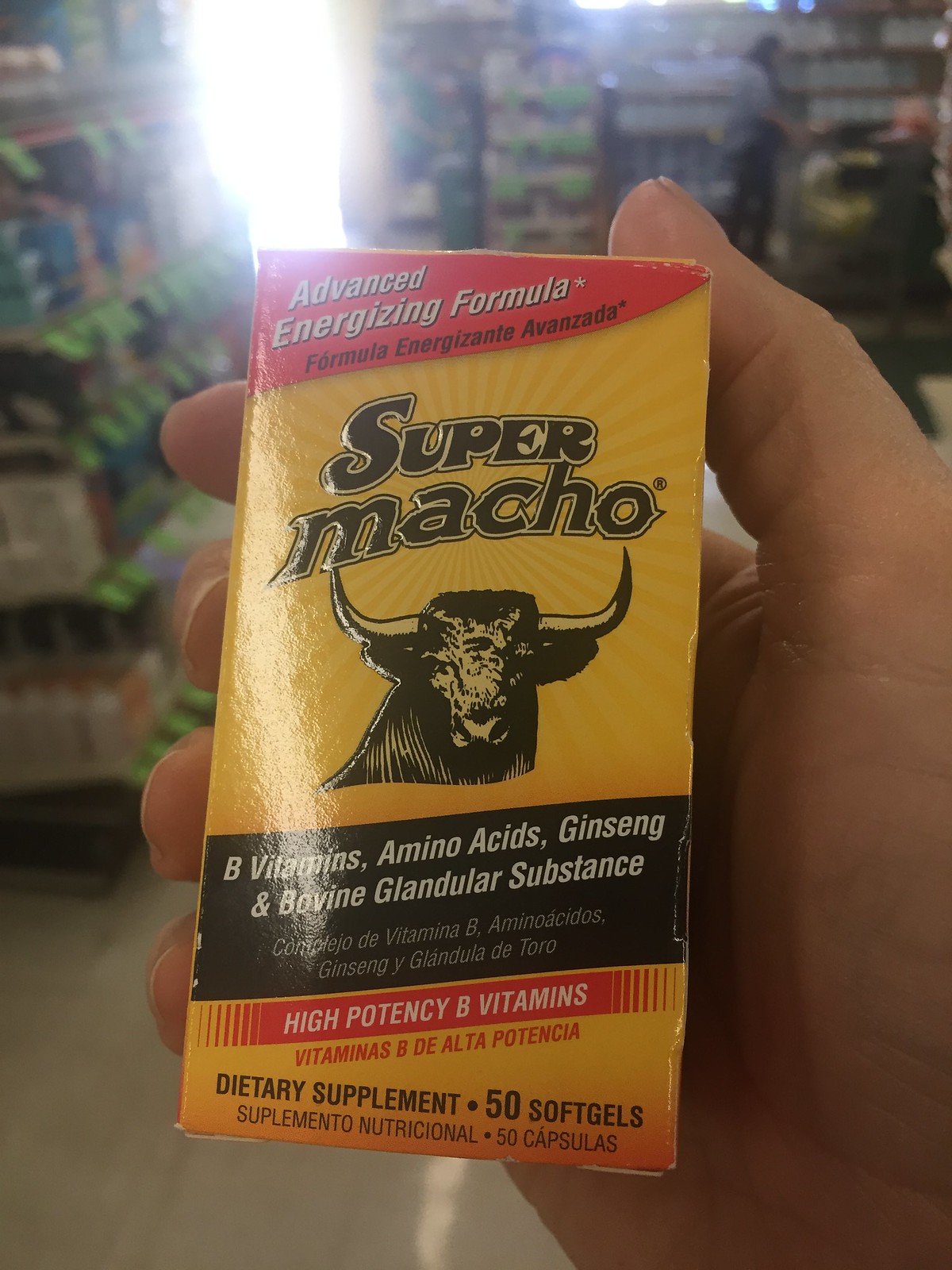The image shows a small rectangular product box held by an open hand, with the thumb positioned on the top right. The box primarily has a yellow background. At the top of the box, on a red background, it says "Advanced Energizing Formula" in white text, followed by the phrase in Spanish - "Formula Energizante von Zappa" marked with an asterisk. Centrally located on the box is the text "SUPER MACHO" in black, with "SUPER" in uppercase and "macho" in lowercase. Below this text is an orange circle with a copyright symbol and a pencil drawing of a bull featuring very long, sharp horns. Underneath the bull illustration, on a black background, it lists ingredients: "B vitamins, amino acids, ginseng, and bovine glandular substance." Further down, the box states "high-potency B vitamins, dietary supplement, 50 soft gels," some of which is also translated into a foreign language. The background of the image reveals the interior of a store with shelves visible.